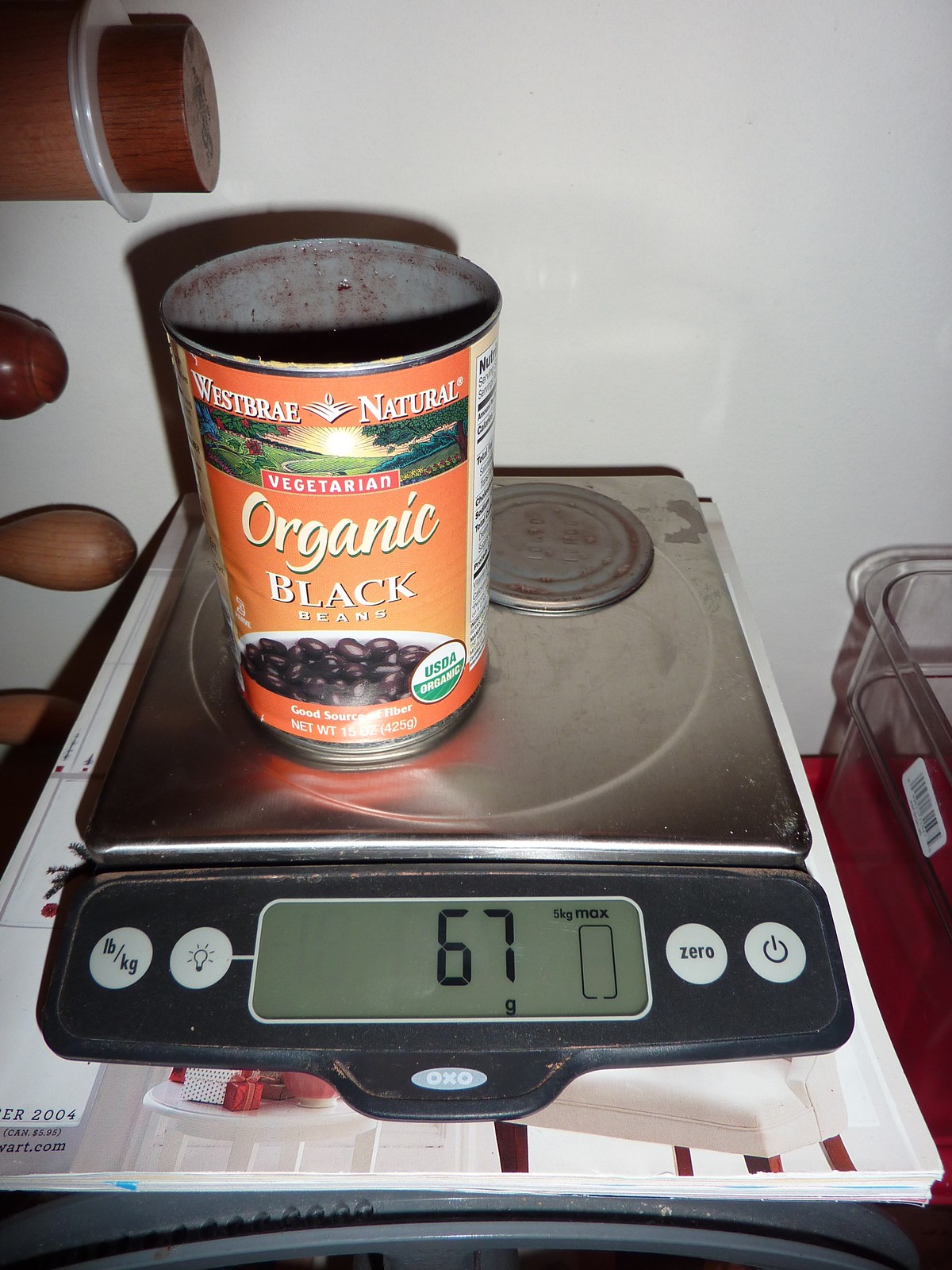This indoor photograph captures a stainless steel food weighing scale positioned on a dark red kitchen countertop. The scale, manufactured by OXO, features a stainless steel plate and a digital display reading "67 grams" (with a small "g" below the "7"). The control panel is black, with four white buttons on both the left and right sides; the left buttons are labeled with an "LB/kg" weight option and a light icon, while the right buttons include a circle for zeroing the scale and a power button. Resting on the scale is an open can of West Bray Natural Vegetarian Organic Black Beans, which has an orange label showcasing an image of black beans on a white plate and a USDA Organic sign. The can's lid is removed, exposing the debris of the beans and sauce inside. The scale sits atop some magazines, in front of a white wall. To the left, there's the end of what appears to be rolling pins, and to the right, a clear plastic container. The image is set against a kitchen backdrop, highlighting a frequently used, slightly dirty scale.